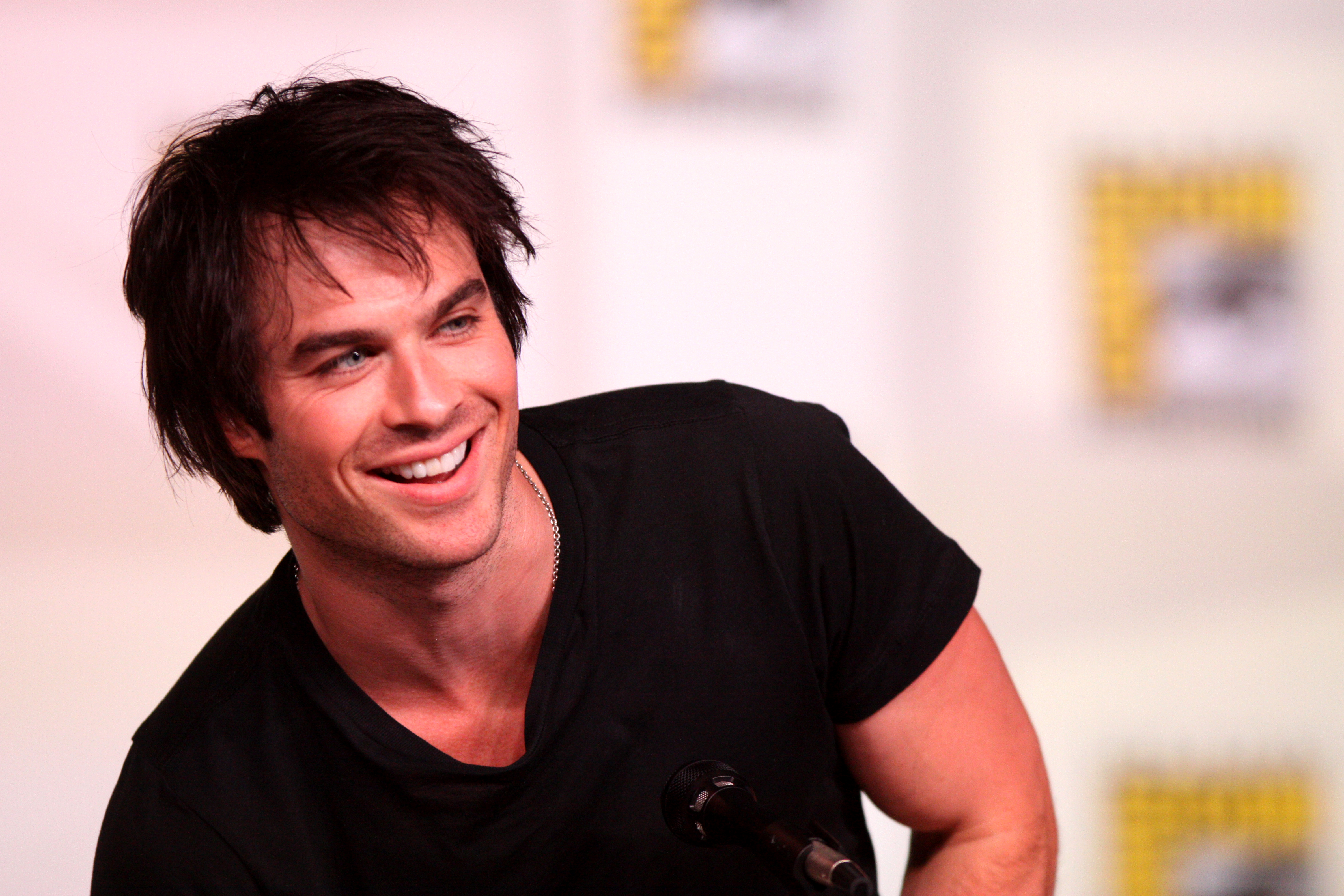This image captures Ian Somerhalder at Comic-Con, leaning slightly to his left. The background features a blurry white backdrop with the yellow Comic-Con insignia repeated across it. Ian is sporting a messy, short, whiskey-brown hairstyle and has light blue eyes that are looking off to the right. He is wearing a black t-shirt paired with a thin silver chain necklace, mostly tucked under his shirt. A subtle five o'clock shadow frames his lips, jaw, and cheeks. His mouth is open in a broad smile, showing his upper set of teeth. A black and silver microphone is positioned in front of him, adding to the candid atmosphere of the photo. He has a visibly defined arm and medium bushy brown eyebrows, contributing to his rugged appearance.